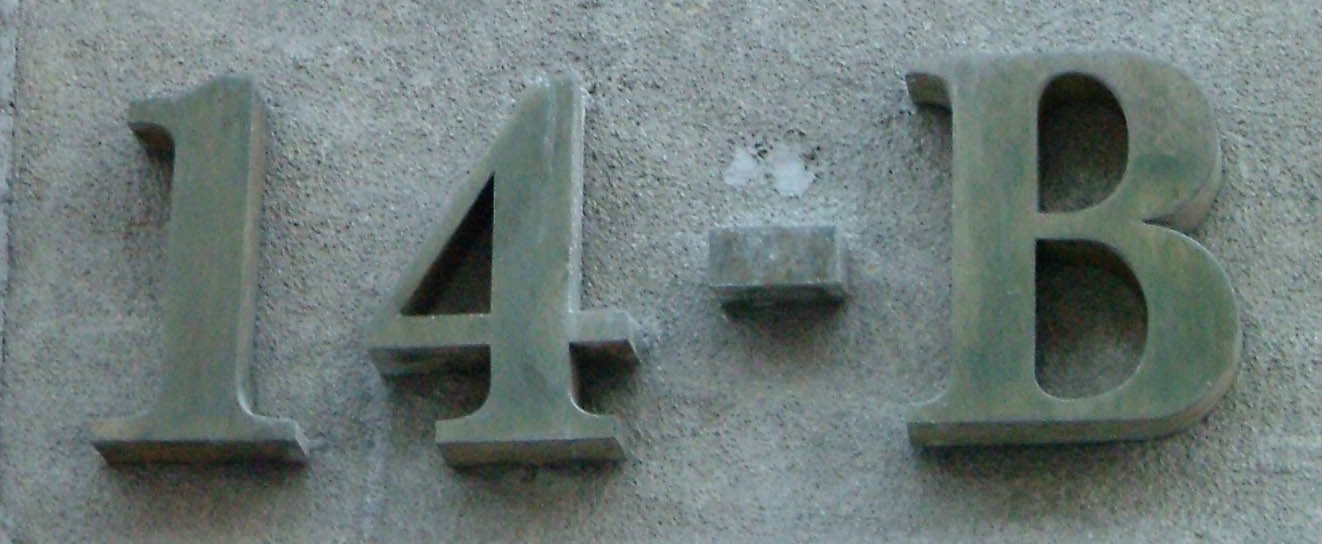The image depicts a close-up view of a sign mounted on the textured, greyish-green wall of a building. The sign features bold, 3D characters in a serif font that read "14-B". These characters are slightly worn and have a tarnished appearance, with a grey color brushed with hints of blue-green, possibly due to discolouration or moss. The background of the image, which could either be a wall or a floor, has a rough texture, and there appears to be a lighter, faded area just above the horizontal slash between the numerals. Additionally, a vertical line extends downward from the lower left edge of the numeral 4, indicating wear on the background. The photo is in narrow landscape mode, emphasizing the sign's details while cropping out extraneous surroundings.